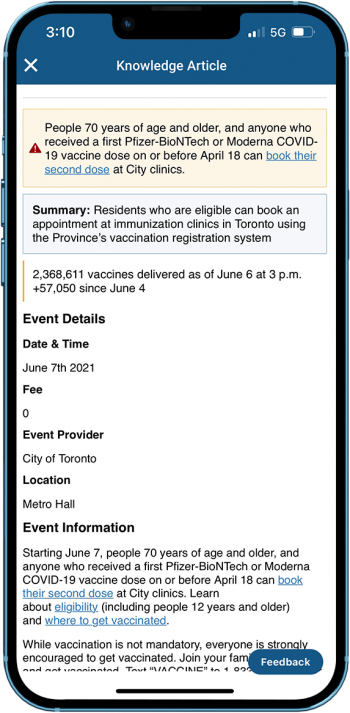A detailed and cleaned-up caption for the mock-up image described:

---

The image is a meticulously detailed mock-up of a smartphone screenshot. The smartphone is encased in metal, with the camera positioned at the top. At the top of the screen, a blue status bar stretches across the width, displaying the time as 3:10, a signal strength of two out of four bars, 5G connectivity, and a battery level at approximately 60%. 

Following this status bar is a header that reads "Knowledge Article," with an "X" button beside it for closing the article. 

Below the header, an alert panel is prominently positioned, displaying an exclamation mark inside a red triangle, indicating an important message. The alert states: “People 70 years of age and older and anyone who received the first Pfizer BioNTech or Moderna COVID-19 vaccine dose on or before April 18th can book their second dose at city clinics.”

A clickable green link follows this statement, directing users to book their second dose appointments.

Beneath the alert panel is another section labeled “Summary,” explaining that residents eligible for the COVID-19 vaccine can book an appointment at immunization clinics in Toronto using the province's vaccination registration system.  

Directly below, a statistic is presented: “2,368,611 vaccines delivered as of June 6th at 3 p.m., 57,050 since June 4th.”

Further down, detailed event information includes:
- **Taking Time:** June 7th, 2021
- **Fees:** Zero
- **Event Provider:** City of Toronto
- **Location:** Metro Hall
  
It reiterates the event information, emphasizing that the booking is for the second vaccine dose.

At the bottom of the screen, there is a blue button labeled “Give Feedback,” providing users with an option to share their thoughts or concerns.

---